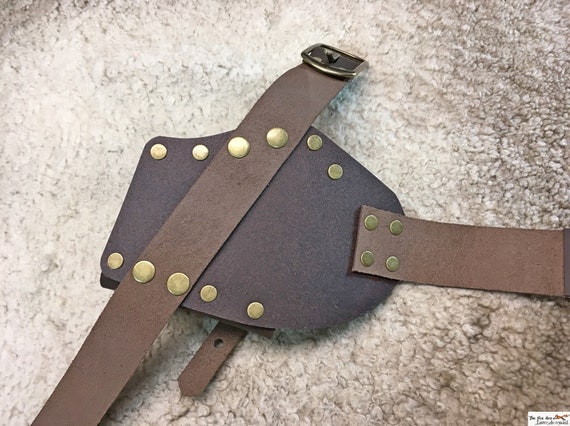The image features a complex arrangement of leather items, prominently including a medium brown leather belt with a small metal buckle, paired with darker brown leather components. The assemblage is held together by approximately 16 circular, gold-colored rivets of varying sizes. The main section consists of an elongated rectangular leather piece, with additional straps and belts hanging off the side and traversing across the top. A notable feature includes a small hole in one of the bottom middle straps. The entire setup is placed on a dark-colored, white carpet that appears somewhat unappealing but soft in texture. In the lower right corner, there is a small, unreadable rectangle with black text, potentially indicating more information about the items, suggesting it might be part of a sales display.